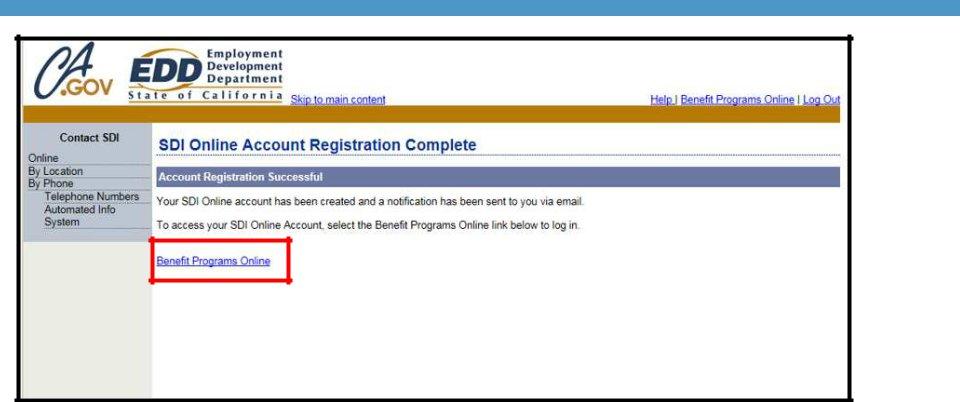The screen features a long light blue horizontal line at the top. Below it, there is a black-outlined square containing the text "ca.gov" and "EDD" in blue. Surrounding this square is a circle in a burnt orange color, accompanied by the text "Employment Development Department, State of California."

Directly beneath this, in blue lettering, it says "Skip to Main Content," with options to the right reading "Help," "Benefit Programs Online," and "Logout." Further down, there's a gray box displaying various contact options: "Contact SDI Online by Location," "by Phone Number," "Telephone Numbers," and "Automated Info System."

To the right, bold blue text reads "SDI Online Account Registration Complete," followed by a blue rectangle stating "Account Registration Successful." Below this, in black lettering, it announces, "Your SDI Online Account has been created and a notification has been sent to you via email." 

To access their SDI Online Account, users are prompted to "select the Benefit Programs Online link below to log in." At the bottom, there's a red square featuring a white background, and in the center, the text "Benefit Programs Online" appears in blue lettering, underlined by a blue line.